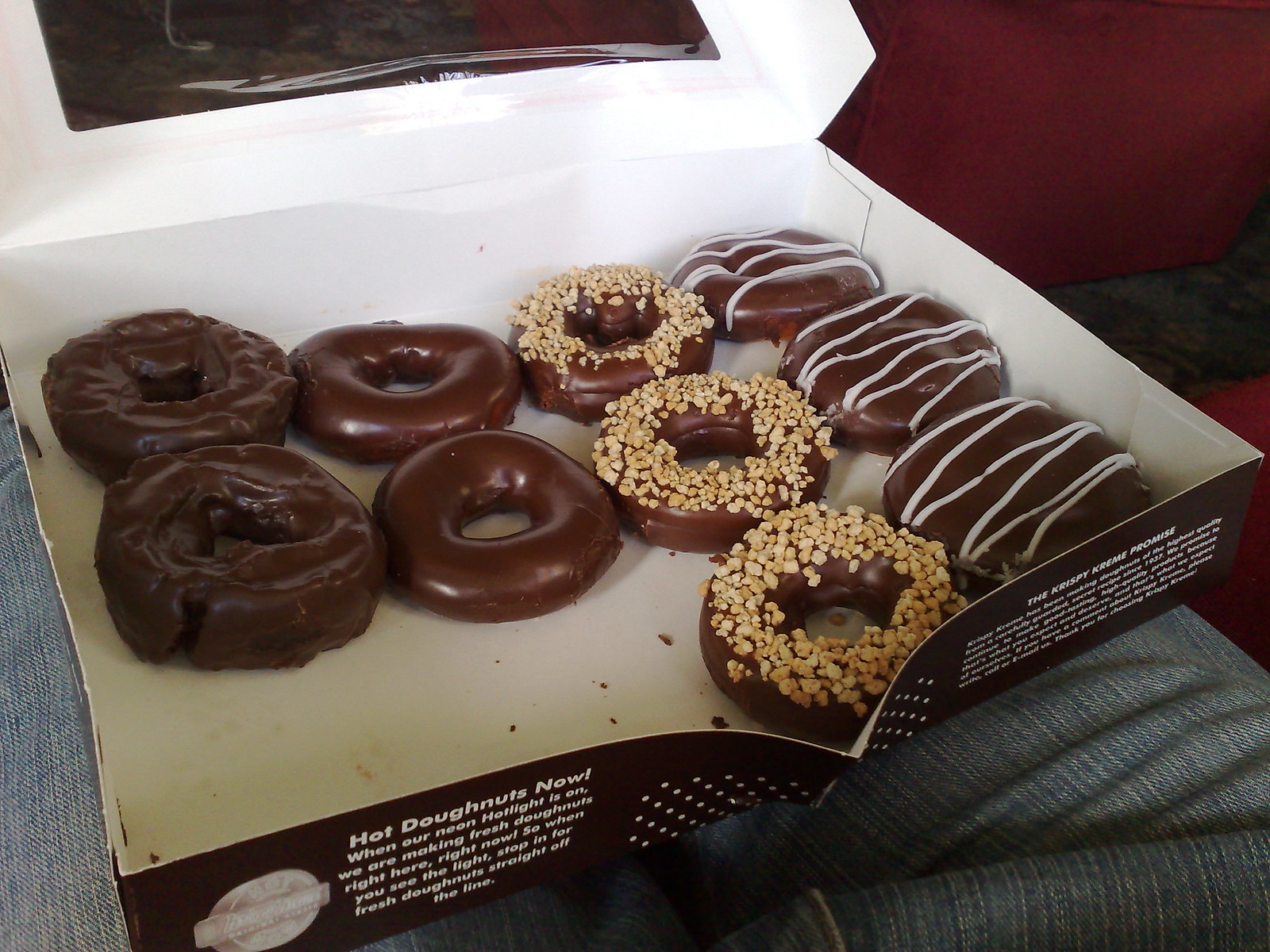This image captures a close-up view of a partially-open Krispy Kreme doughnut box resting on a man's lap, who is wearing light blue jeans. The box, which is rectangular and has a chocolate-colored exterior with white lettering and the Krispy Kreme logo on the bottom left, originally held a dozen doughnuts but now contains ten. The interior of the box is white, and the top features a transparent cellophane lid.

Inside, the doughnuts are neatly organized into three rows. The row on the far right features three filled doughnuts, each completely covered in chocolate with a white icing zigzag pattern. The next row to the left has three standard chocolate-covered doughnuts sprinkled with chopped nuts. The following row consists of two regular chocolate doughnuts, and finally, on the far left, there are two chocolate cake doughnuts. The setting appears to be on gray upholstery, possibly a car seat, and the overall scene suggests the doughnuts were freshly made, indicated by text on the box stating "Hot Doughnuts, Now" when the light is on.